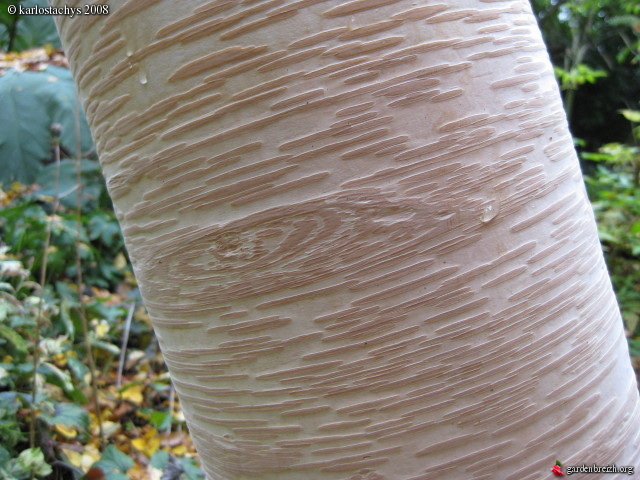In this detailed outdoor image, the focal point is a diagonally positioned tree trunk, prominently occupying around 75-80% of the frame. The bark of the tree is primarily a pale, whitish color with raised, textured areas in varying shades of light brown. These raised sections give the trunk a textured appearance, interrupted by droplets of water, enhancing its naturalistic feel despite appearing almost artificial, as if the bark has been stripped in places. The backdrop features a rich tapestry of nature, including green, yellow, and brown leaves, interspersed with sticks and possibly small trees, painting a vivid forest scene. In the top left corner, bold text reads "Karlotzky's 2008," and in the bottom right, the website "gardenbrzosek.org" is visible. The colors across the image range from browns and tans to greens, blacks, yellows, and oranges, adding depth and vibrancy to this serene natural setting.